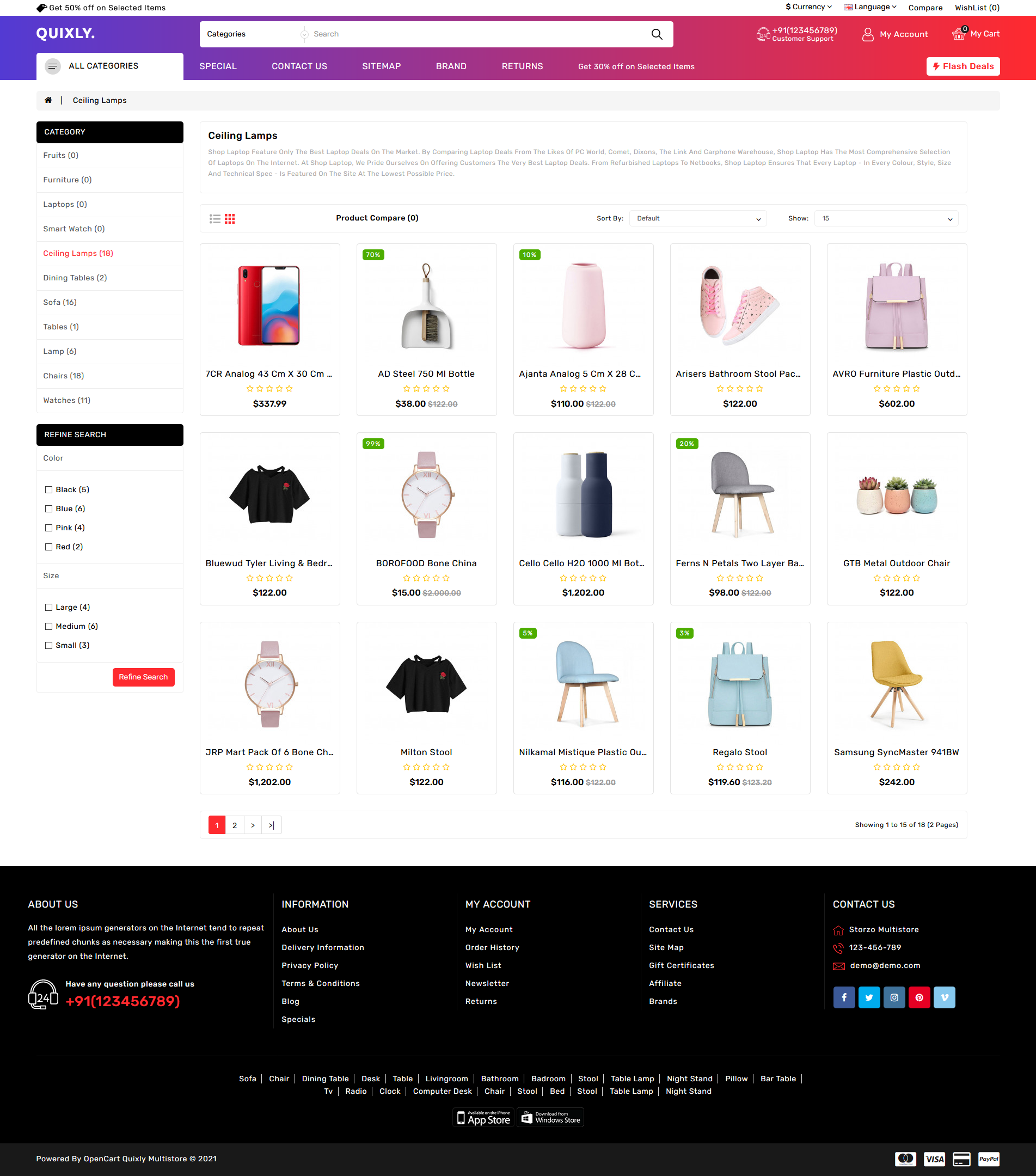Explore amazing deals and discounts! In the top left corner, there’s a bright banner announcing "Get 50% off on select apps." You’ll also notice options for currency selection, language settings, comparing items, adding to your wishlist, navigating through different categories, and a comprehensive search feature. Below that, icons representing various item quantities are displayed: 9, 1, 1, 2, 3, 4, 5, 6, 7, 8, 9.

Moving to the right, a prominent rectangle highlights "Flash Deals." This section is accompanied by links to all categories, special offers, curated content, segments, and brand-specific returns. Another deal banner offers "Get 30% off on select items" against a vibrant red background.

The column on the far left categorizes various items such as fruits, furniture, laptops, smartwatches, ceiling lamps, dining tables, sofas, tables, lamps, chairs, and watches. Below this, a black rectangle provides a refined search option based on color (choices include black, blue, pink, and red) and size (large, medium, small). 

A red button highlights the "Refined Search" for ceiling lamps, offering the best deals from leading brands. Featured is the Alexa PC World’s Comet Dixon Ceiling Lamp (7Cr analog, 43cm x 30cm) priced at $337.90, a significant markdown from its original price of $750,000. Other highlighted items include dustpans, gentle analogs, risers, bathroom stools, and more. 

Each product is labeled accurately, displaying categories like Afro furniture, plastic outdoor beds, Tyler living room items, blue word bags, bear-themed shirts, and a Burr bone China Celo watch (Celo H20, $1,000). Additionally, find furniture options such as pillows, tooler bars, TTP metal outdoor chairs, and more. Shop now for unbeatable deals and refine your search to find the best products tailored to your needs!